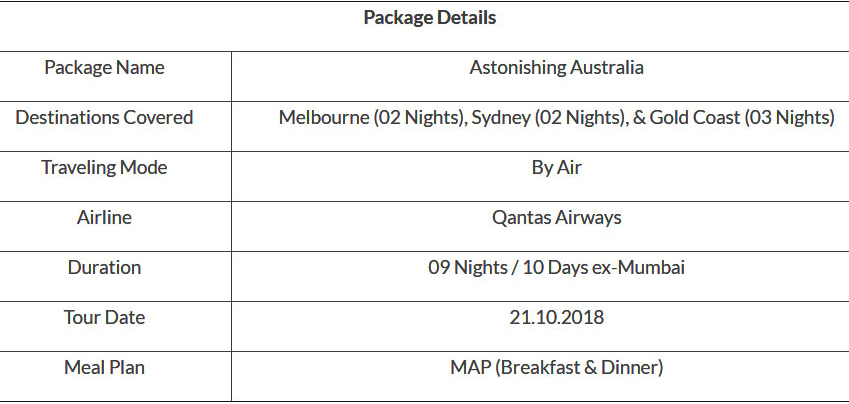This is a receipt, possibly sent via email, presented as a straightforward printout without any web page elements. It appears to be an invoice for a travel package titled "Astonishing Australia," detailing the following:

**Package Details:**

- **Package Name**: Astonishing Australia
- **Destinations Included**: 
  - Melbourne: 2 nights
  - Sydney: 2 nights
  - Gold Coast: 3 nights
- **Mode of Travel**: By air, via Qantas Airways
- **Trip Duration**: 9 nights and 10 days
- **Departure Location**: Mumbai
- **Tour Dates**: October 21, 2018
- **Meal Plan**: MAP (Modified American Plan) including breakfast and dinner

No pricing details are provided in the document. The receipt is formatted in a basic, black-and-white spreadsheet style, with a clear, organized layout. The package name and its description are separated by a vertical line down the middle, effectively dividing the content into two clear sections, resembling a typical invoice setup.